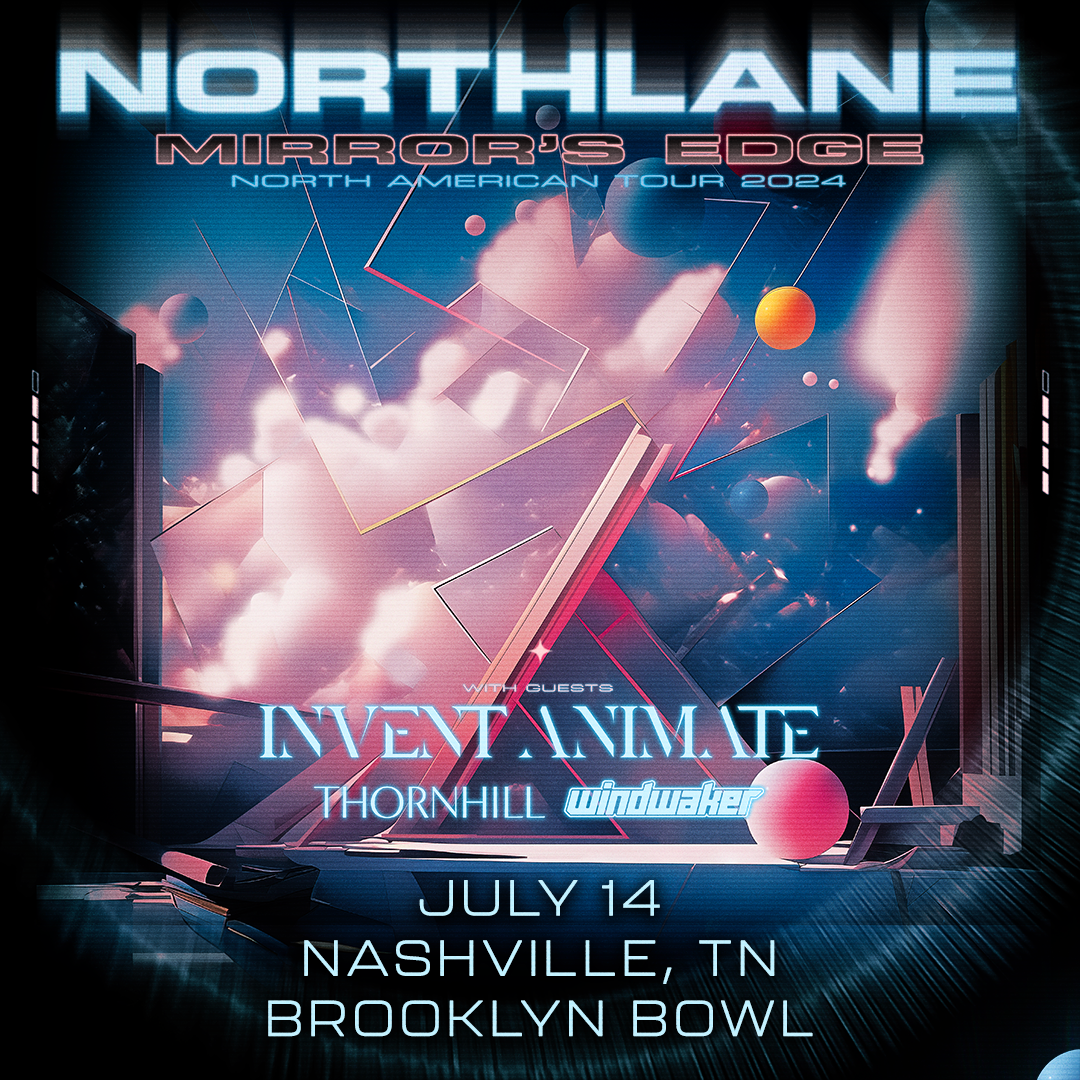The poster features a striking black background with a series of detailed and vibrant graphic elements. At the top, the text "North Lane" is prominently displayed in a white font with a slightly blurry effect and an outline, immediately catching the eye. Directly below this, the words "Mirror's Edge" appear in brown writing, and beneath that, the phrase "North American Tour 2024" is in a bold blue font.

The middle section of the poster showcases an abstract design rich in blue tones with white clouds, creating a sense of depth and dimension. Several colored spheres are dispersed throughout this section: a large blue sphere under the word "tour," smaller ones scattered near "North Lane," and additional black, pink, orange, and purple spheres. Notably, a large pink sphere and an orange one are positioned at the bottom, accompanied by elements resembling broken glass and mirror frames, adding texture and intrigue. 

The lower portion of the poster lists additional details in light blue text, including the names of guest bands: Invent, Animate; Thornhill; and Wind Waker. It culminates in the event specifics, stating "July 14th, Nashville, Tennessee, Brooklyn Bowl," in a striking light blue font.